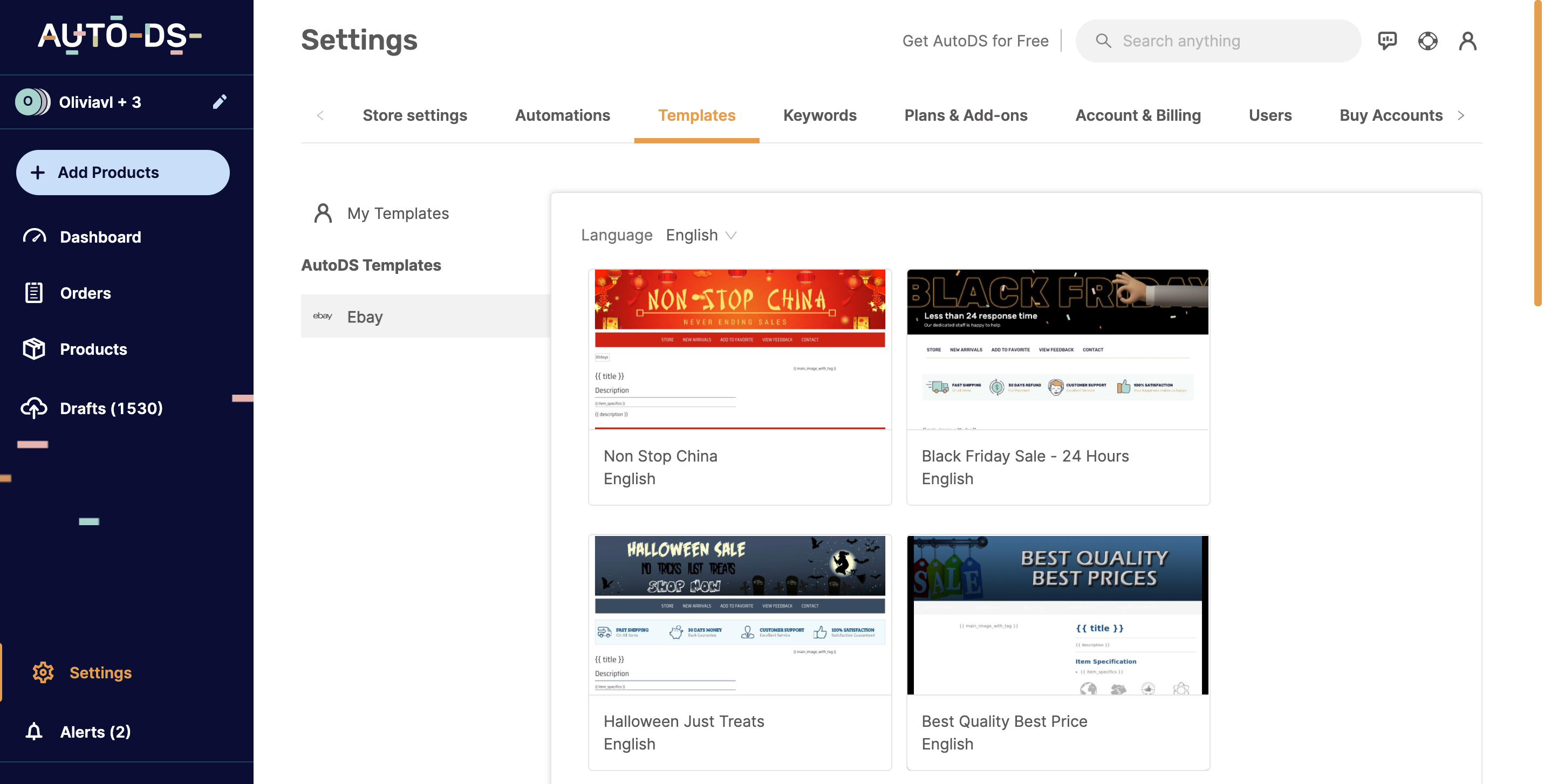In this image, we observe a comprehensive settings menu on a web page, showcasing a well-organized layout. On the left side, there is a vertical, rectangular menu with a contrasting black background. At the top of this menu, it prominently displays "Auto DS." Just below it, the user "Olivia VL plus 3" is listed. Following this, there is a button labeled "Add Products," and further down, we find additional navigation options such as "Dashboards," "Orders," "Products," and "Drafts."

Shifting our focus to the right side of the screen, the main section has a clean, white background with the word "Settings" written in bold black text at the top. Adjacent to this, on the extreme right, a search bar is available, inviting the user to "Search anything." Below the search bar, a series of buttons provide access to various settings categories: "Store Settings," "Automations," "Templates," "Keywords," "Plans and Add-ons," "Account and Billing," "Users," and "Buy Accounts."

Further down, there is a dedicated section labeled "My Templates," featuring a subsection for "Auto DS Templates." Displayed here are several templates tailored for different retail occasions, including "Non-stop China," "Black Friday Sale," "Best Quality, Best Price," and "Halloween is Just Treats." This image captures a user-friendly interface designed to facilitate efficient navigation and management of e-commerce functionalities.